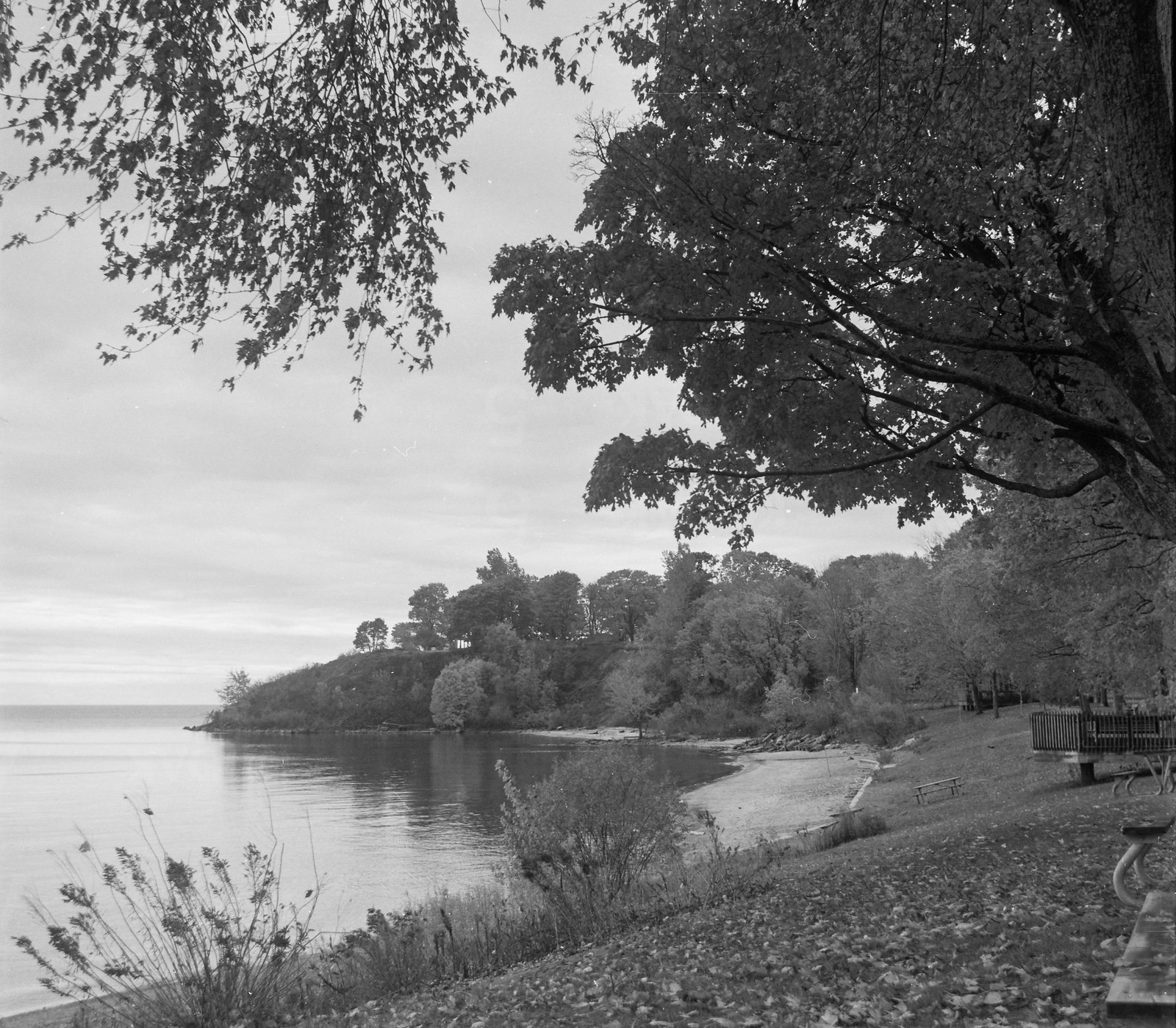This black and white photograph captures a serene lakeside scene. The image, slightly more vertical than horizontal, presents a tranquil lake occupying the left side, with a U-shaped cove or small bay that creates a peaceful inlet. Sand stretches between the calm water and a grassy bank to the right. Trees with their branches gently overhang the upper left and upper right corners, casting a natural frame around the scene. In the foreground, several plants and bushes spread from the bottom left toward the center, adding texture to the grass hill that slopes gently toward the beach.

A wooden bench or perhaps a dock area stands in the lower right, partially hidden by overhanging tree branches. This bench, alongside what seems to be wooden decking, offers a restful viewpoint over the calm waters. The sky, heavy with gray clouds, blankets the scene in a muted, contemplative atmosphere. Distantly, land covered with trees forms natural borders to the lake, with a hill running down to the water's edge. This photograph beautifully captures the peaceful coexistence of natural elements in a grayscale spectrum, highlighting the interplay of water, sand, grass, and foliage under an overcast sky.